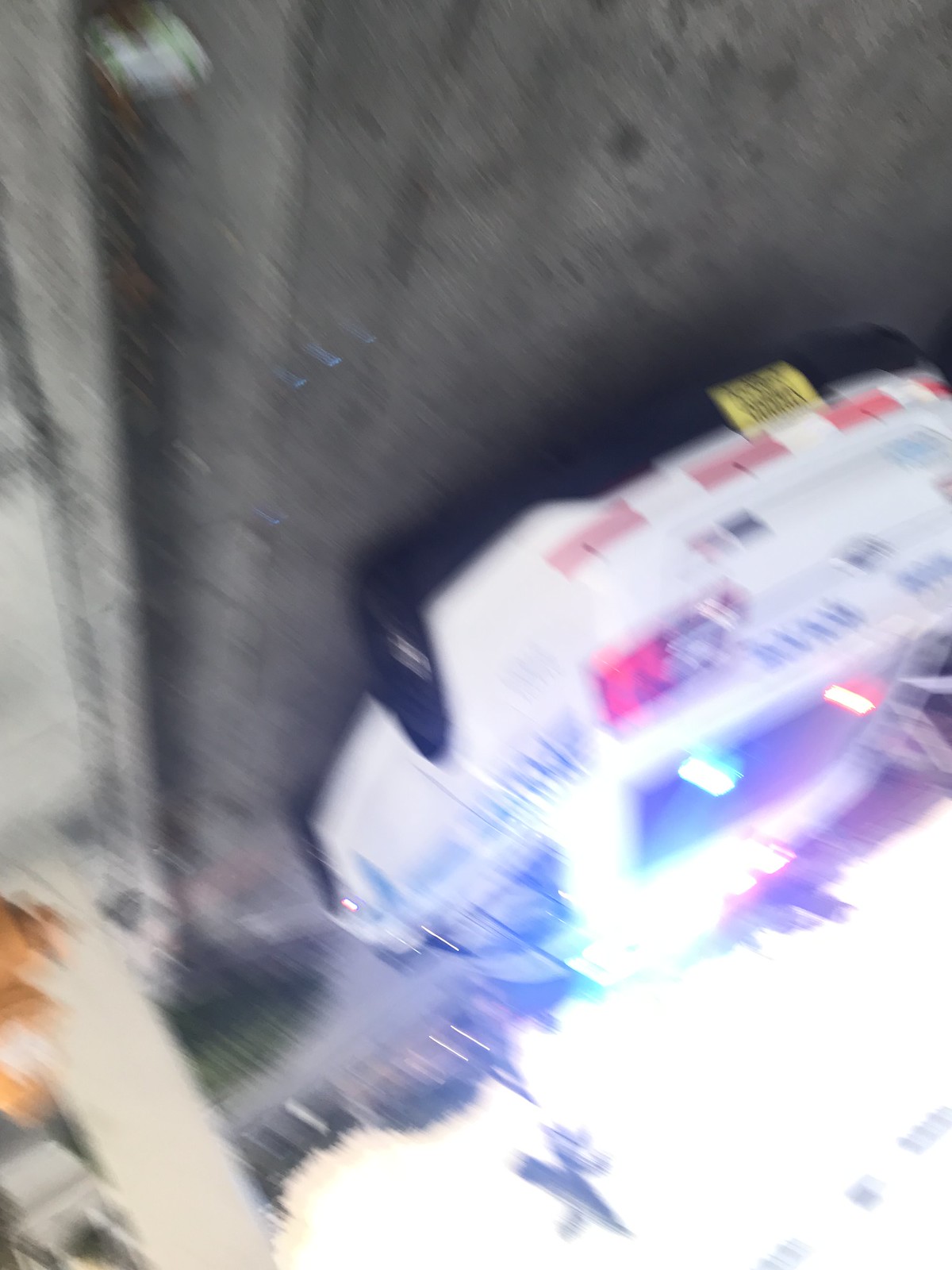An upside-down photograph captures what appears to be a police car stationed on the side of a road. The vehicle is predominantly white with blue writing on its rear and side, indicating its official capacity. On the passenger door, there is a distinctive blue medallion symbol. The car's license plate is yellow, mounted on the back end of the vehicle, and directly above it are four red rectangles. When the image is oriented correctly, a yellow fire hydrant and a sturdy pillar can be seen to the right of the vehicle, bordered by some lush green bushes or trees, adding depth and context to the urban setting.